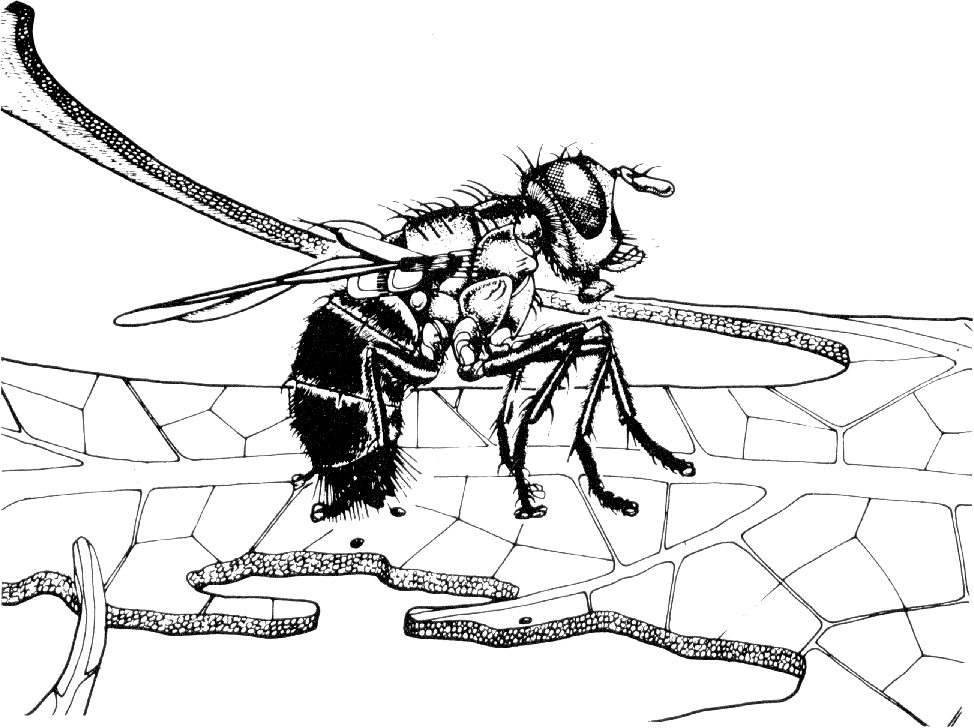This black-and-white line drawing depicts a large housefly, viewed from the side and positioned towards the right. The housefly is detailed with several legs extended out front, a pair of big eyes, and downward-pointing mouthparts. Its wings are not spread out but folded and oriented towards the left. The fly is perched on a ground made up of irregularly shaped stones or bricks, shaded in black with white highlights, giving the impression of a cracked sidewalk. The entire drawing is set against a stark white background, emphasizing the intricate details of the large insect without any additional elements like borders, text, plants, or human activity.